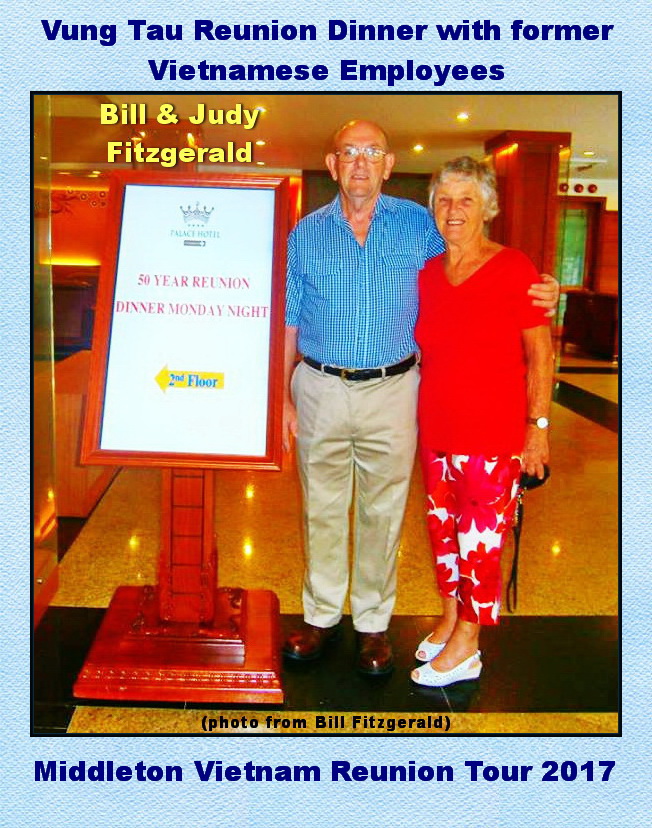This tall, rectangular image features a captioned, framed photograph with a light blue textured frame, wider at the top and bottom than at the sides. At the very top, it boldly reads in navy blue font: "Vung Tau Reunion Dinner with Former Vietnamese Employees," and underneath, in the same font, "Middleton Vietnam Reunion Tour 2017." 

The photograph captures an older couple—Bill and Judy Fitzgerald—standing beside a sign in what appears to be a hotel lobby. Bill, on the left, sports a blue checkered button-down shirt, khaki pants, a dark brown belt, and brown shoes. His arm is around Judy, who stands on the right, dressed in a red v-neck shirt and white pants adorned with large red flowers. The sign next to them, in pink font, announces: "50-Year Reunion Dinner Monday Night." 

The detailed caption is further supplemented at the bottom with a note in black font: "Photo from Bill Fitzgerald."